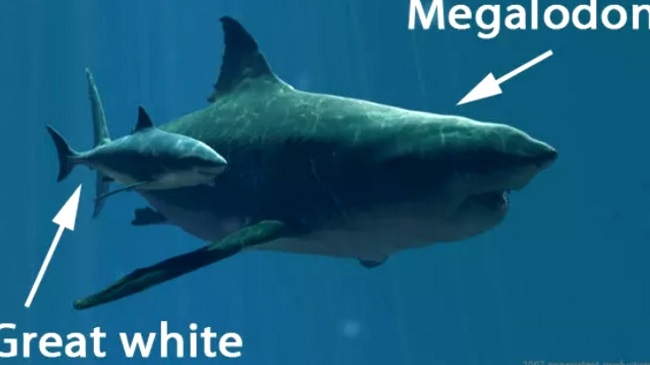In this digitally rendered image, two sharks are shown swimming through a clear blue underwater backdrop. On the left side, a smaller shark, labeled "Great White" with a white arrow pointing towards it from the bottom left, is depicted. This Great White shark has a medium gray body with a lighter white-gray underbelly and a prominent dorsal fin. 

On the right side, towering over the Great White, is a much larger shark labeled "Megalodon." This prehistoric giant is identified by multiple white arrows, one pointing from the top right corner and another from the top left. The Megalodon is about five or six times larger than the Great White, with a body that shades from dark gray to a slightly greenish tint and a similarly lighter underbelly. Its imposing figure has a pointed nose and a partially open mouth, illustrating its massive scale in comparison to the Great White. The depiction serves as a striking visual comparison between the modern-day Great White shark and its extinct relative, the Megalodon.